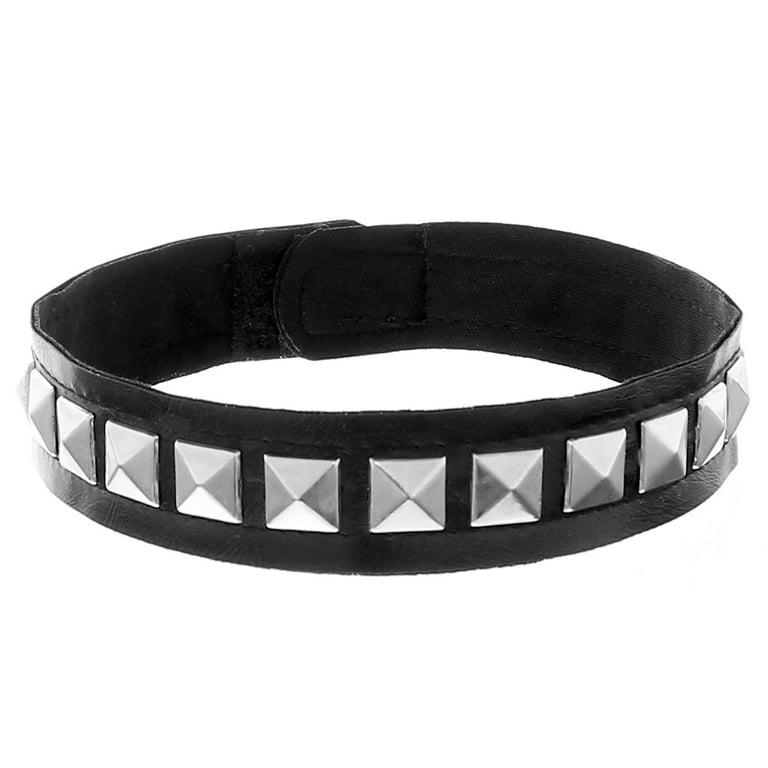The image features a bracelet or belt made of black leather or plastic material on a white background, giving it a floating appearance. The band is about two inches thick and is detailed with metallic pyramid studs, each silver in color, lining the exterior. These studs are square, slightly raised, and divided into a pattern of triangles, resembling two envelopes with touching points. Approximately twenty to twenty-two studs adorn the entire band, with eleven visible on each side. The band is accentuated with thin leather rims at the top and bottom, with visible black stitching. The latch or clasp at the back appears Velcro-like, securing the band.